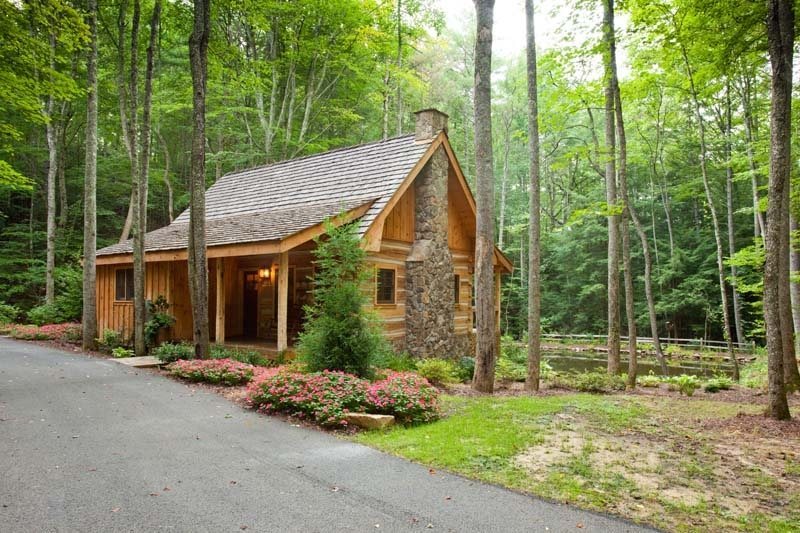The image depicts a small wooden cabin in a lush, green forest during the daytime. The cabin, made entirely of brown timber, features a grey, angled roof and a stone chimney positioned on the center-right side. A covered front porch with a wooden door and beams supporting a canopy faces to the left of the image. Tall and skinny trees with foliage concentrated at the top surround the cabin, contributing to the dense forest setting. In front of the cabin, there is a small garden area with bushes and pink flowers, adding a touch of color to the scene. A cement path extends from the front of the cabin toward the viewer, functioning as a driveway. Additionally, a small pond can be seen behind the cabin, further enriching the picturesque forest environment.